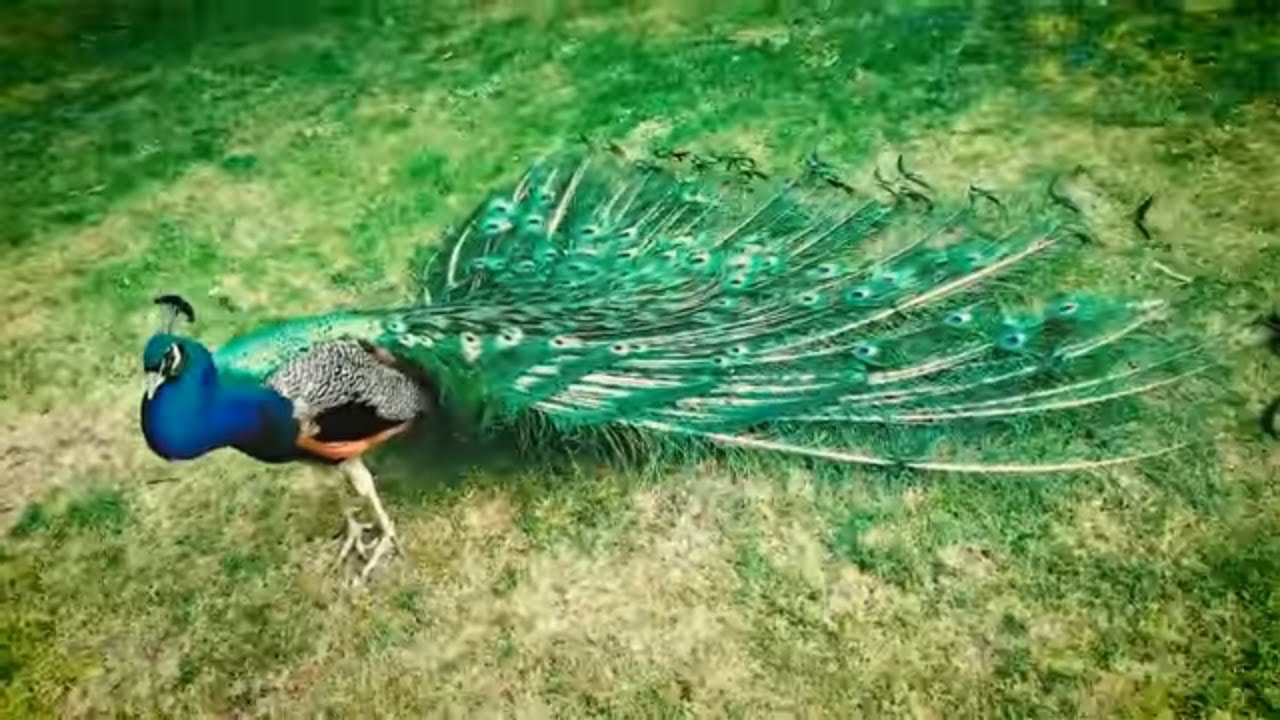In this outdoor image, we see a peacock standing gracefully in a grass field, with her long, green tail feathers laying gently on the ground. The multicolored grass beneath her feet features patches of dry yellow areas as well as healthier dark green sections. The peacock herself is strikingly beautiful, with a vibrant blue neck—a typical color for female peacocks—and a slender body. Traditional black feather details adorn the back of her head, and her body also showcases black and white patterns with hints of orange. Her distinct tail feathers, which feature characteristic eye shapes, are primarily green and subtly interspersed with white, enhancing the overall elegance of her appearance. The peacock is positioned towards the left side of the image, with the cascading length of her stunning tail feathers extending towards the center.